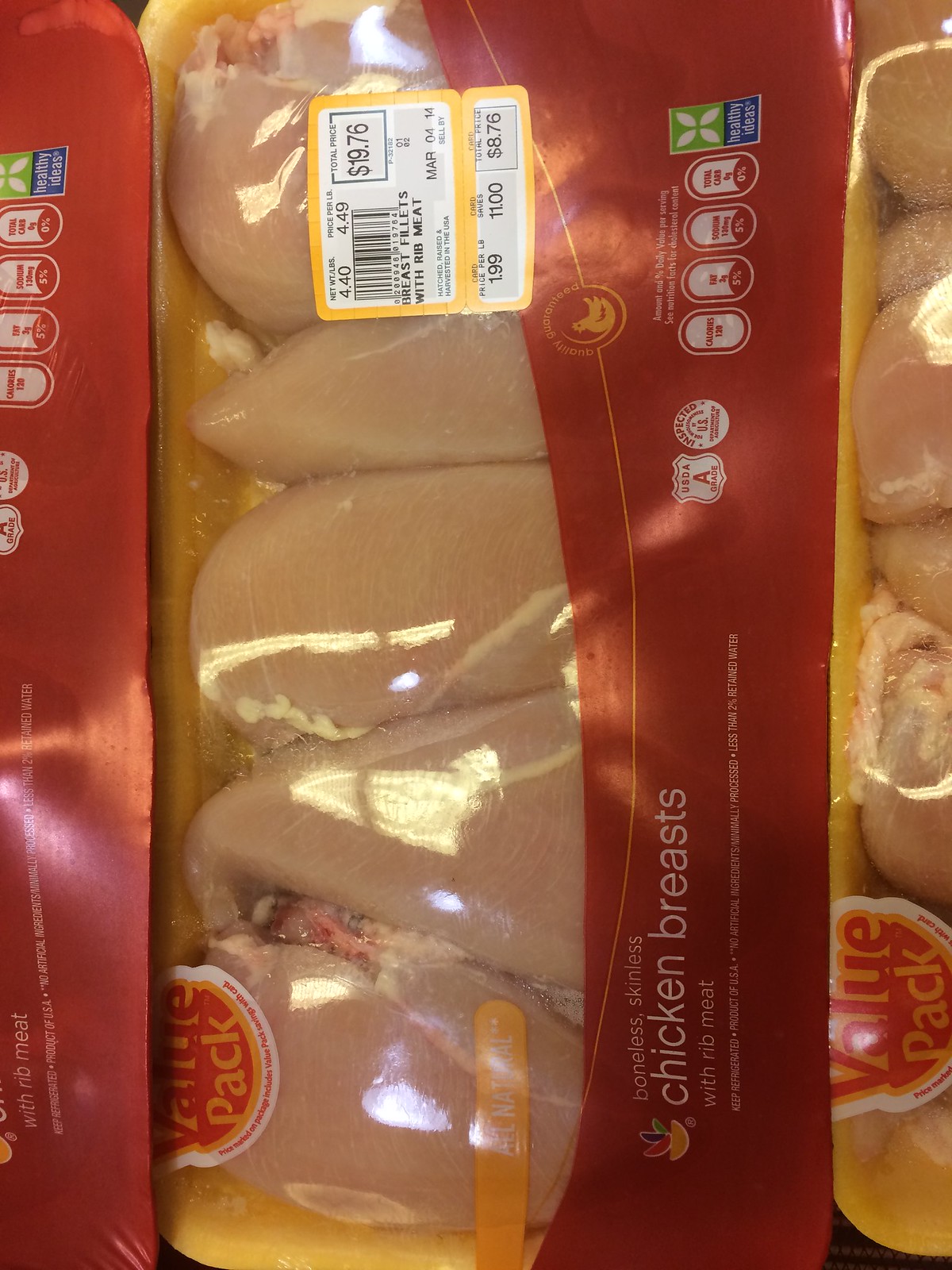A vertically-oriented photo displays a package of boneless, skinless chicken breasts with rib meat, prominently labeled as a "Value Pack." The packaging is clear, revealing approximately six chicken breasts inside, and features a deep burgundy-red background with white text. Key details on the label include the price of $19.76, with the chicken priced at $4.49 per pound and the total package weighing 4.40 pounds. An additional yellow label, possibly with a SKU, highlights more information in black and white text. The setting appears to be within a store cooler, as another partially visible chicken breast package can be seen at the top and bottom edges of the photo.